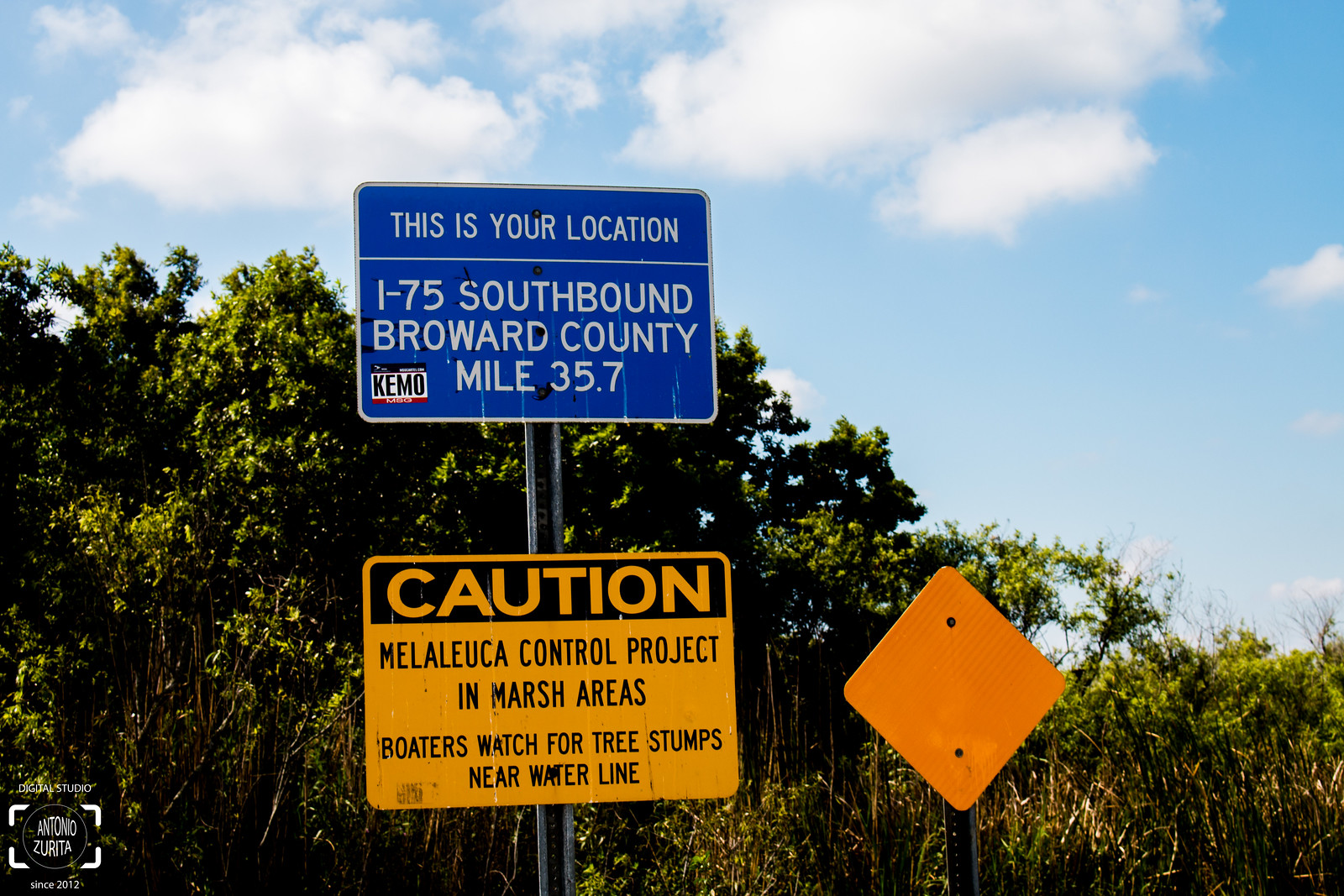The image depicts a bright, daytime outdoor setting with a clear blue sky dotted by a few puffy white clouds. The foreground features a lush, green area filled with trees and brush, occupying the bottom and middle portions of the image. On the left side, there are distinct signs placed on a black post secured by two black bolts. A plain white diamond-shaped sign is prominent. Above it, a blue rectangular sign has white text stating, “This is your location I-75 southbound Broward County mile 35.7,” along with a small sticker bearing the letters "KEMD." Beneath this, a yellow rectangular sign reads, “Caution, Melaleuca control project in marsh areas. Boaters watch for tree stumps near waterline.”